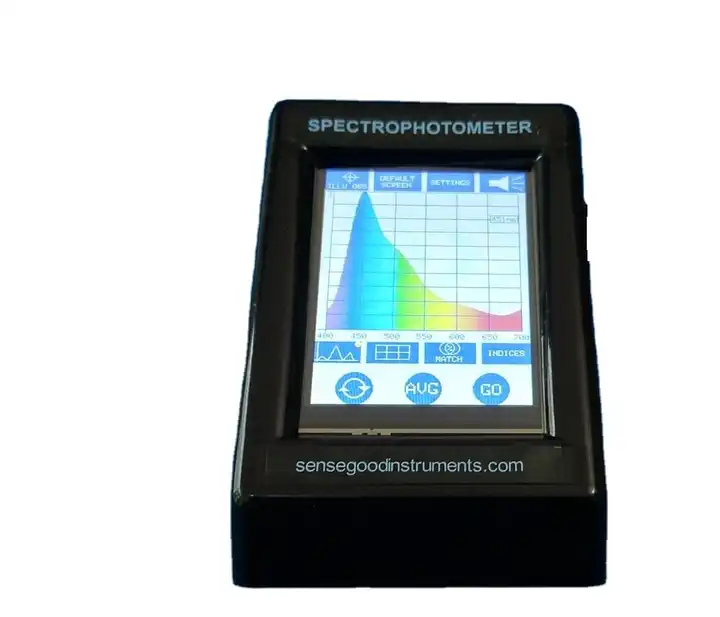This image depicts a black spectrophotometer from GoodSenseGoodInstruments.com, likely dating back to the 1980s or 1990s. Prominently featured on the top of the device is the word 'spectrophotometer,' while the bottom displays the website 'sensegoodinstruments.com.' The device has a small screen bordered by thick, chunky edges and houses several blocky, blue-colored buttons, which offer various functionalities such as graphs, match indices, average, go, settings, and numerous light options. The screen displays a rainbow-colored graph with a gradient that peaks on the left side in purple and gradually slopes down to a hot red on the right. This colorful gradient likely represents a scale of different light wavelengths. The spectrophotometer resembles a credit card machine in size and shape, adding to its robust, retro aesthetic.